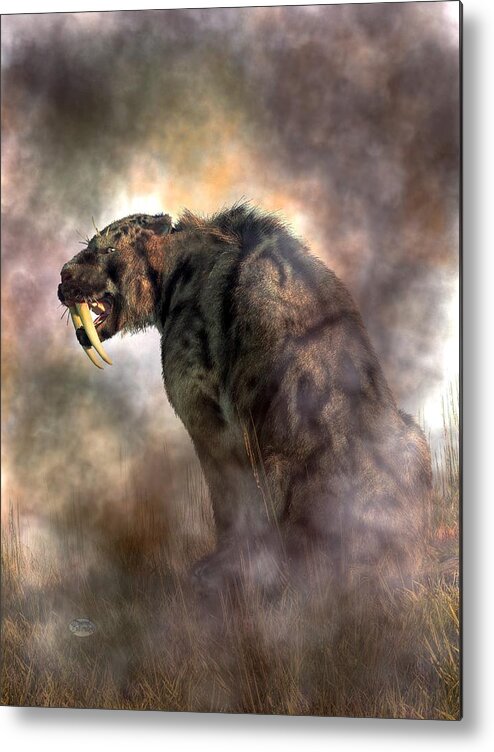The image portrays a detailed painting of a saber-toothed tiger, or saber-toothed cat, imbued with an ancient and almost eerie aura. The animal is depicted sitting amidst tall, dry grass with its muscular forearms resting on the ground. The setting evokes a prehistoric atmosphere, highlighted by a cloudy, foggy background filled with black and gray smoke that swirls around and partially obfuscates the tiger, adding to the painting's mystique. The tiger, with its light brown fur adorned with black stripes, splotches, and hints of gray and reddish-orange on its upper body and head, looks formidable and predatory. Its head is turned slightly to the left, glaring menacingly with a single visible eye. Its mouth is partially open, prominently displaying its massive saber-like canines, similar to tusks, contributing to its ferocious appearance. The artwork has a signature located at the bottom left in an oval, adding a final touch of authenticity to the painting. The overall scene exudes a haunting and primeval essence, capturing the power and mystery of this extinct predator.